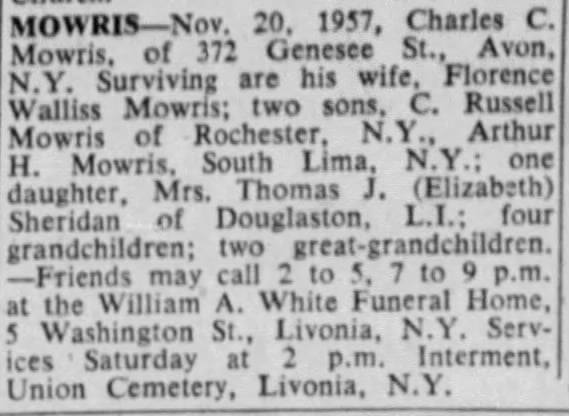The image shows a newspaper obituary for Charles C. Maury, who passed away on November 20th, 1957, and resided at 372 Janice Street, Avon, New York. He is survived by his wife, Florence Wallace Maury, two sons, C. Russell Maury of Rochester, New York, and Arthur H. Maury of South Lima, New York, and one daughter, Mrs. Thomas J. Elizabeth Sheridan of Douglaston, Long Island. He also leaves behind four grandchildren and two great-grandchildren. Friends may call from 2 to 5 p.m. and 7 to 9 p.m. at the William A. White Funeral Home, located at 5 Washington Street, Livonia, New York. The funeral service is scheduled for Saturday at 2 p.m., with interment to follow at Union Cemetery in Livonia, New York. The obituary is simple and concise, typical of its publication in a newspaper, though the exact year of printing is not specified.